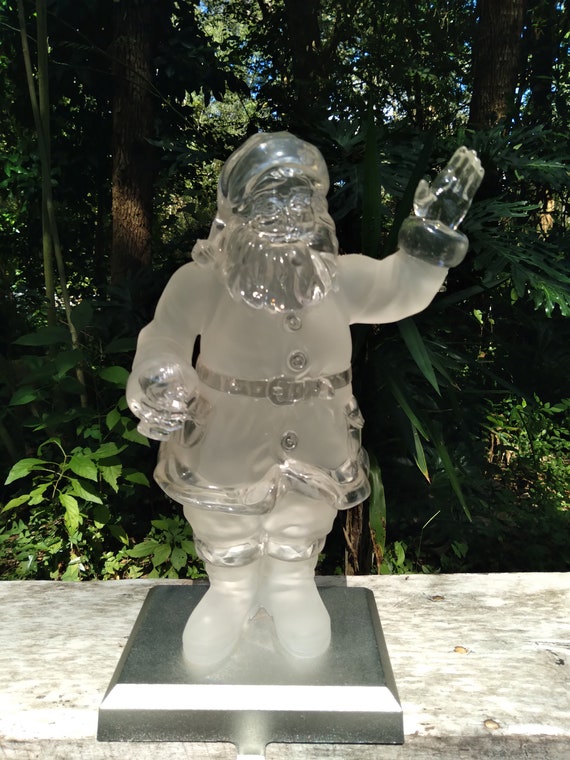This photograph captures a detailed statue that resembles a jolly Santa Claus, characterized by his big beard, boots, and iconic Santa outfit with a large belt. Santa is depicted waving with his left hand while holding something indeterminate in his right. The statue, notable for its semi-transparency and frosty appearance, suggests it might be sculpted from ice, though it could also be made from clear plastic or glass. It is prominently displayed on a silver-colored metal base, which itself rests on a sturdy, gray stone wall. The backdrop of the scene features lush greenery with tree trunks, bushes, ferns, and glimpses of the blue sky peeking through the leaves, indicating it is set in a garden environment. The photograph is taken in a portrait orientation, emphasizing the vertical arrangement of the elements.